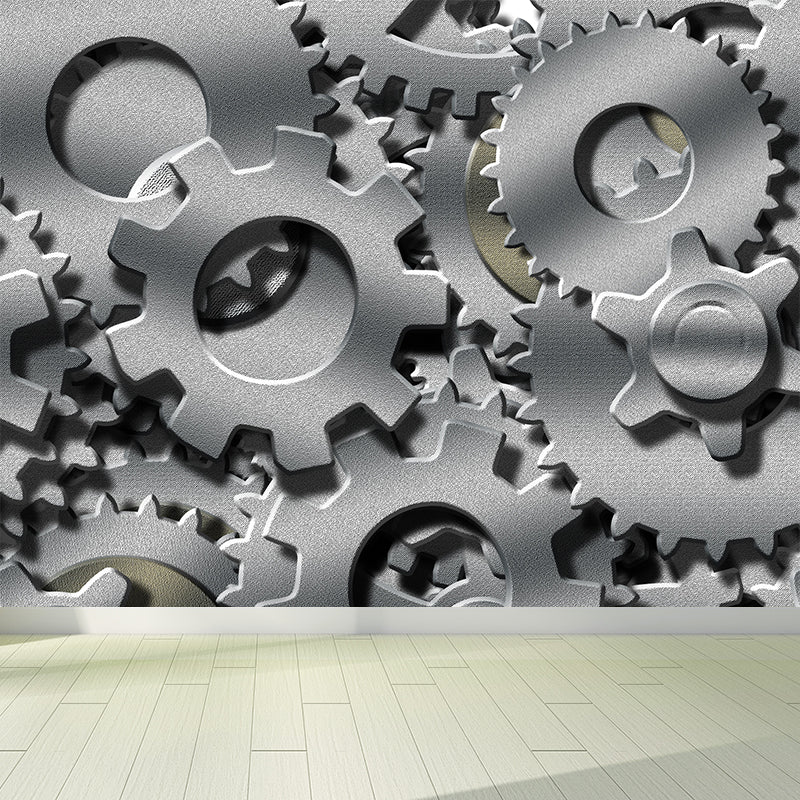In the image, we see a meticulously rendered computer illustration of numerous silver metal gears, layered intricately on a wall. These gears vary in design—some feature block-like, chunky spokes, while others possess slimmer, more numerous spokes. The gears interlock seamlessly, creating the illusion of a smoothly functioning machine. The wall itself is accentuated by careful shadowing, enhancing the 3D effect of the otherwise 2D painted design. All this is set against a backdrop of a light-colored wood laminate floor, approximating a white or light brown hue, accompanied by a clean white baseboard at the bottom. The overall composition conveys a sense of perpetual motion and intricacy, despite its static nature.